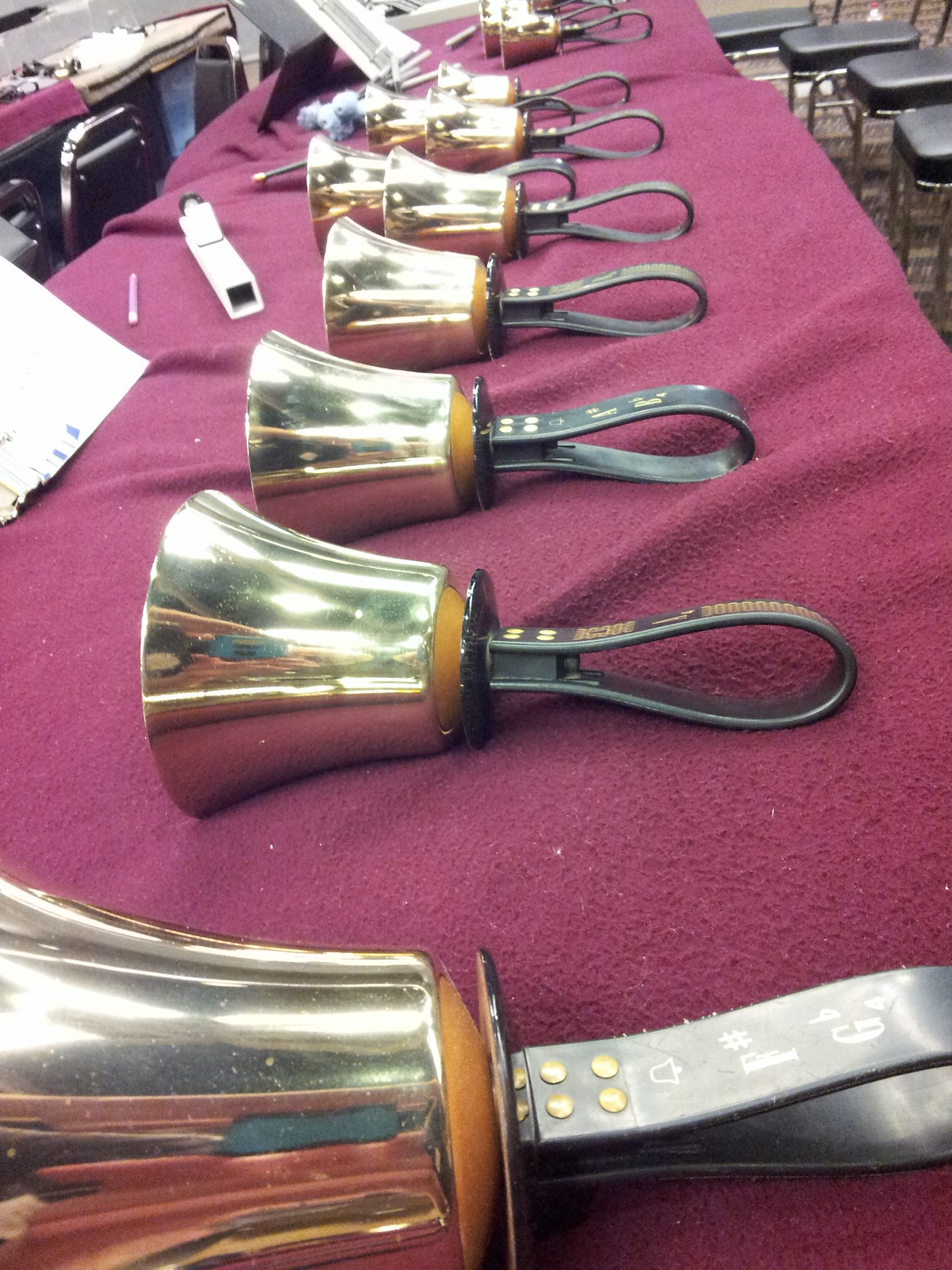The photograph showcases a meticulously arranged line of at least 11 brass-colored bells on top of a table draped with a dark crimson, felt-like blanket. The bells, all largely identical, feature black, oval-shaped handles attached by four brassy studs. With the angle of the photograph, the nearest bell is prominently labeled "F sharp G flat," while the remaining bells are not clearly labeled but presumably have different notes. The table setting contrasts notably against the rich, deep red fabric below. The scene includes additional black chairs with silver legs visible on the right, and more chairs paired with an indistinct collection of instruments on another table to the left. The arrangement and details evoke a sense of careful preparation, possibly for a musical performance.